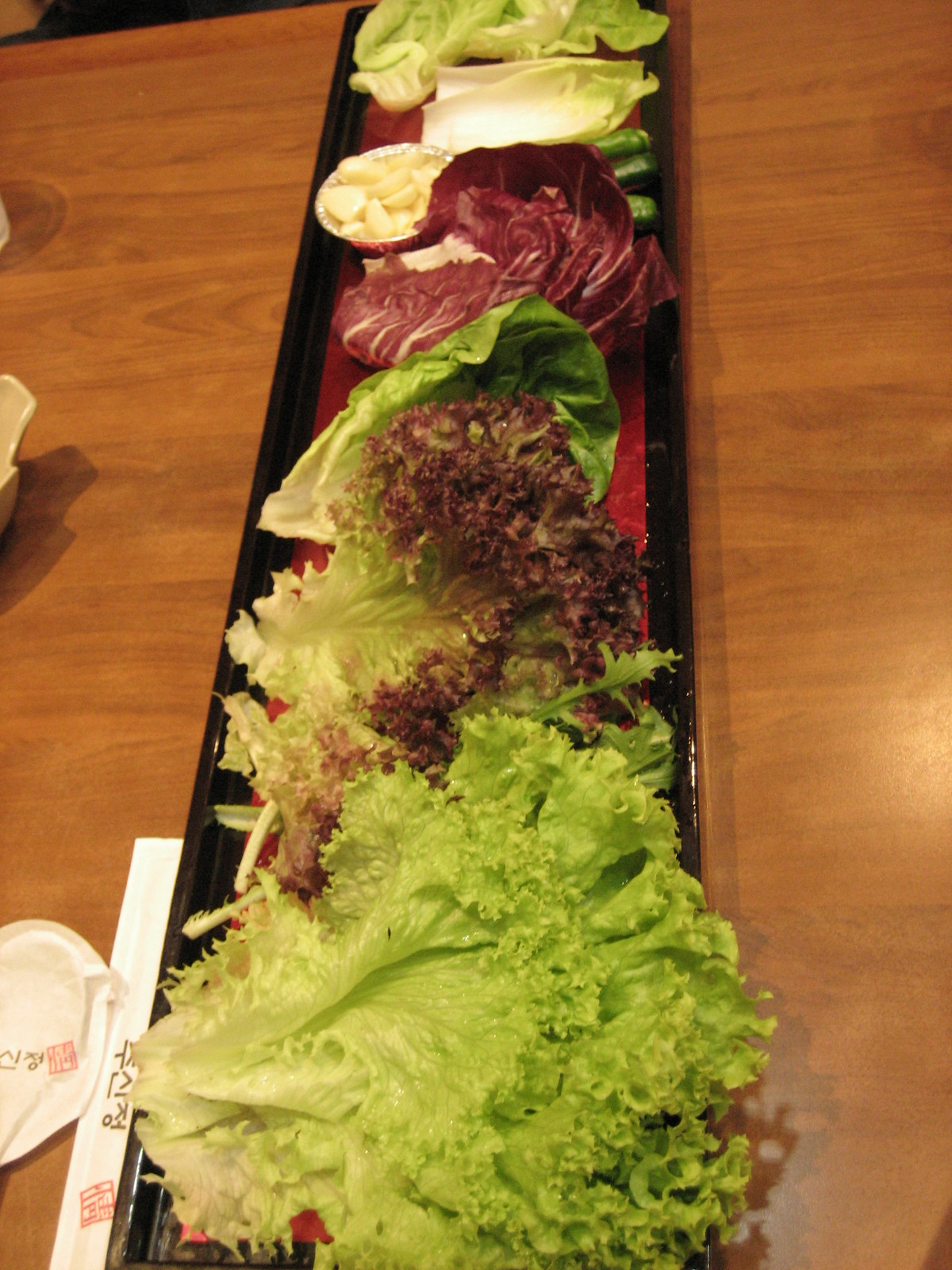The image captures a reddish-gold wooden table viewed from above, featuring a visually striking arrangement. Central to the composition is a long, flat tray with a black edge and a deep red center. This tray spans the table and is meticulously adorned with a variety of vegetables, prominently featuring several types of lettuce and leafy greens, including romaine lettuce and purple cabbage, arranged artfully from one end to the other. The vibrant display of greens and purples creates a lush, appealing contrast with the tray's red background. To the lower left, a small white glass bowl contains water chestnuts or a similar item, complementing the fresh produce. Nearby, a white wrapper with Chinese lettering and a set of plastic-wrapped chopsticks add an authentic culinary element to the scene, hinting at a meal experience that may involve wrapping ingredients in the leafy greens. A wrapped spoon is also visible, adding a touch of functionality to the elegant setting.